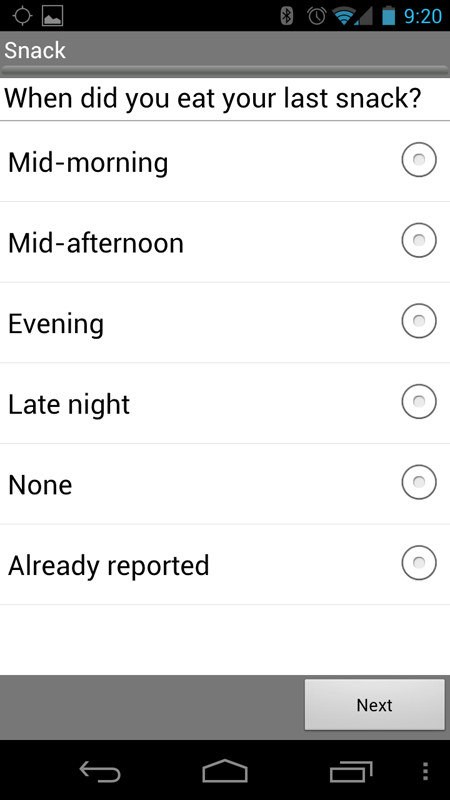Screenshot of a phone display showing a questionnaire related to snack times. At the top of the screen, a timestamp reads "9:20." The main text of the page asks, "When did you eat your last snack?" followed by six options:

1. Mid-morning
2. Mid-afternoon
3. Evening
4. Late night
5. None
6. Already reported

Currently, no option has been selected. At the very bottom of the screen, there is a "Next" button. Below this button, the footer contains four icons: one for navigating backwards, a home icon, an icon displaying two stacked rectangles, and an icon with three vertically stacked dots.